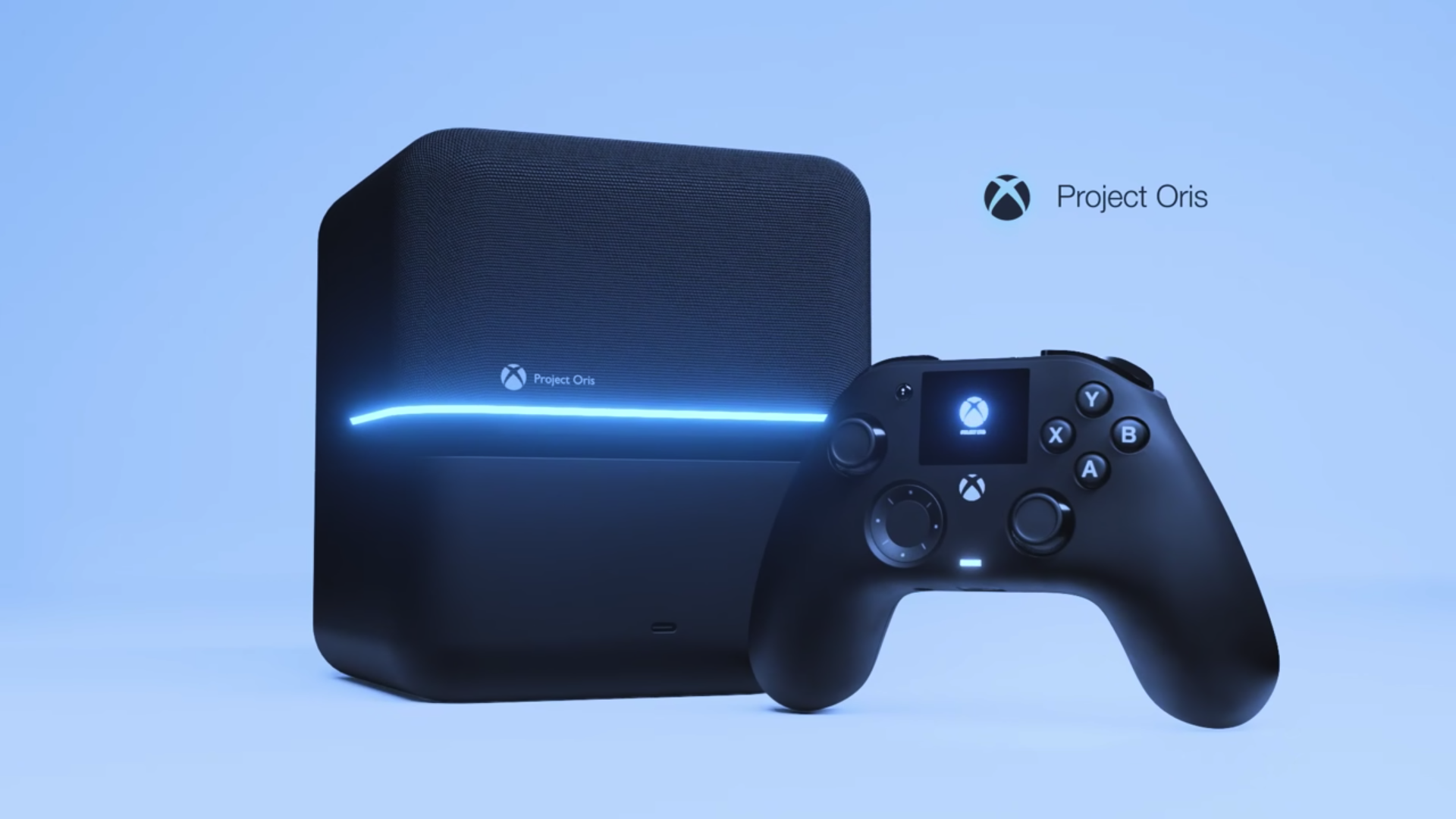The image appears to be an advertisement with a light blue background, presented in a horizontal rectangle. At the center, prominently featured, are two black objects. On the left is a black square or cube with a line of light blue light running horizontally across its middle. Above this line, there is an Xbox logo and the text "Project AORUS."

To the right of the square object is a classic Xbox-style controller. It's black, equipped with the Y, X, A, and B buttons on the right side, a directional pad in the lower left, and joysticks positioned in the upper left and lower right. In the middle of the controller, there is a small rectangular screen displaying the Xbox logo. Above the two main objects, on the right side of the image, there is another Xbox logo accompanied by the words "Project AORUS" in blue lettering.